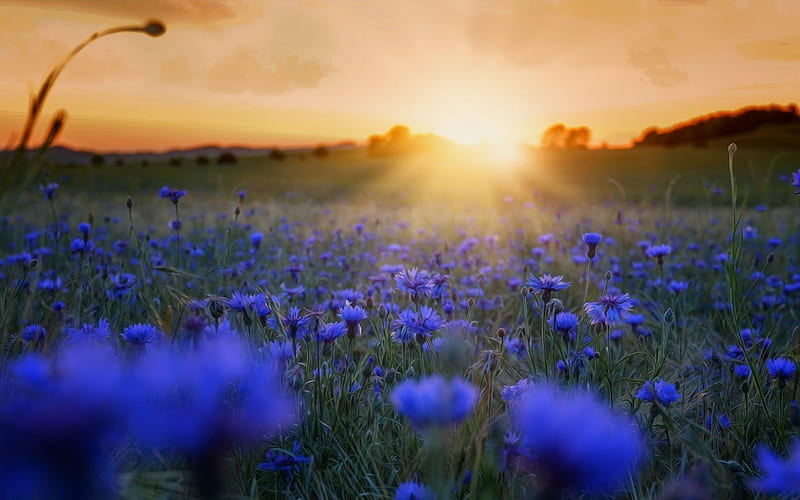This captivating nature landscape photo showcases a serene meadow teeming with deep blue flowers, possibly cornflowers or a similar species. In the immediate foreground, some flowers are so close to the camera that they're intentionally blurred, contributing to the immersive depth of the scene. There's a distinctive hanging flower on the left side, which resembles a dandelion. As our gaze extends towards the horizon, the sun is either rising or setting, casting a weak yet enchanting orange hue across the sky and allowing brilliant yellow beams to light up the upper portion of the image. Silhouettes of treetops and gentle hills frame the background. The overall impression is one of untouched beauty, with no signs of human presence, capturing the tranquil essence of a sun-dappled meadow or fields awaiting new crops. The perspective suggests the photographer is lying forward in the meadow, drawing us even closer into this tranquil, picturesque moment.